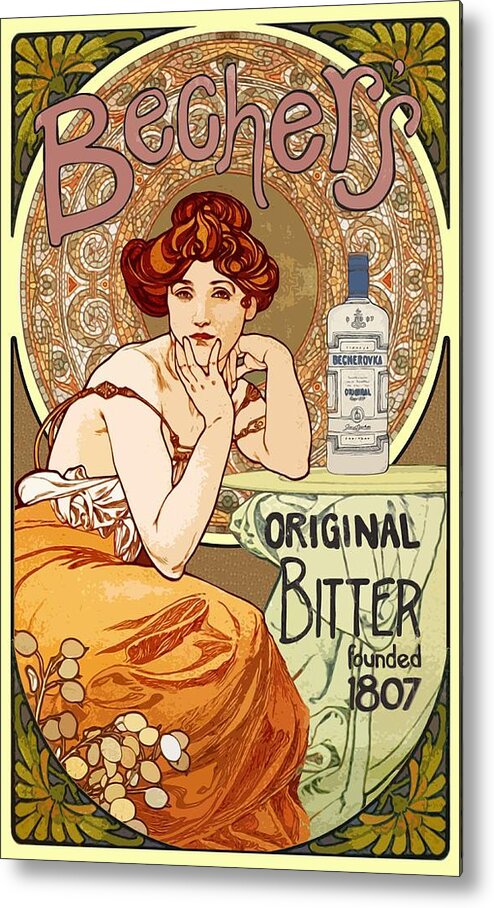The image is a tall, rectangular, vintage-style poster with distinct Art Nouveau elements reminiscent of Alphonse Mucha's work. It features a woman with vibrant, ornate red hair piled atop her head, leaning her left elbow on a beige table. Her right hand, forming a V-shape with her fingers, thoughtfully supports her chin. She is dressed in an intricate orange dress and is depicted with a pale complexion.

The background showcases elaborate, circular, and floral patterns in gold and silver, adding to the old-fashioned aesthetic. At the top of the poster, the word "Bechers" (or possibly "Beechers"), written in inflated, wavy, 70s-style pink lettering, forms part of the vintage charm. 

On the table to the woman's right, there's a white bottle with a blue top, labeled "Becherovka," containing the text "Original Bitter Founded 1807" in the lower right quadrant, indicating it's an advertisement for this liquor. Overall, the poster blends ornate art with a sense of nostalgia, emphasizing the woman’s graceful pose and the decorative, flowing elements surrounding her.